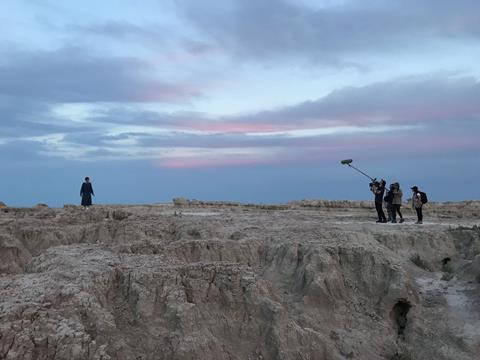The image captures a desolate, rocky desert landscape with a light brown-grey terrain that appears dry and craggy. In the distance, there's a small group of people, seemingly a film crew, equipped with a large camera and a long pole-mounted microphone. On the left side of the image, a person dressed in a long-sleeved, black dress stands on one of the larger rocks, gazing away from the camera, their arms relaxed at their sides. The scene is set against a backdrop of a dusky sky, streaked with shades of pink, suggesting the time might be early morning or late evening. The rough terrain features distinct peaks, hollows, and grooves, resembling a hilltop or canyon rim, further adding to the isolated nature of the setting.